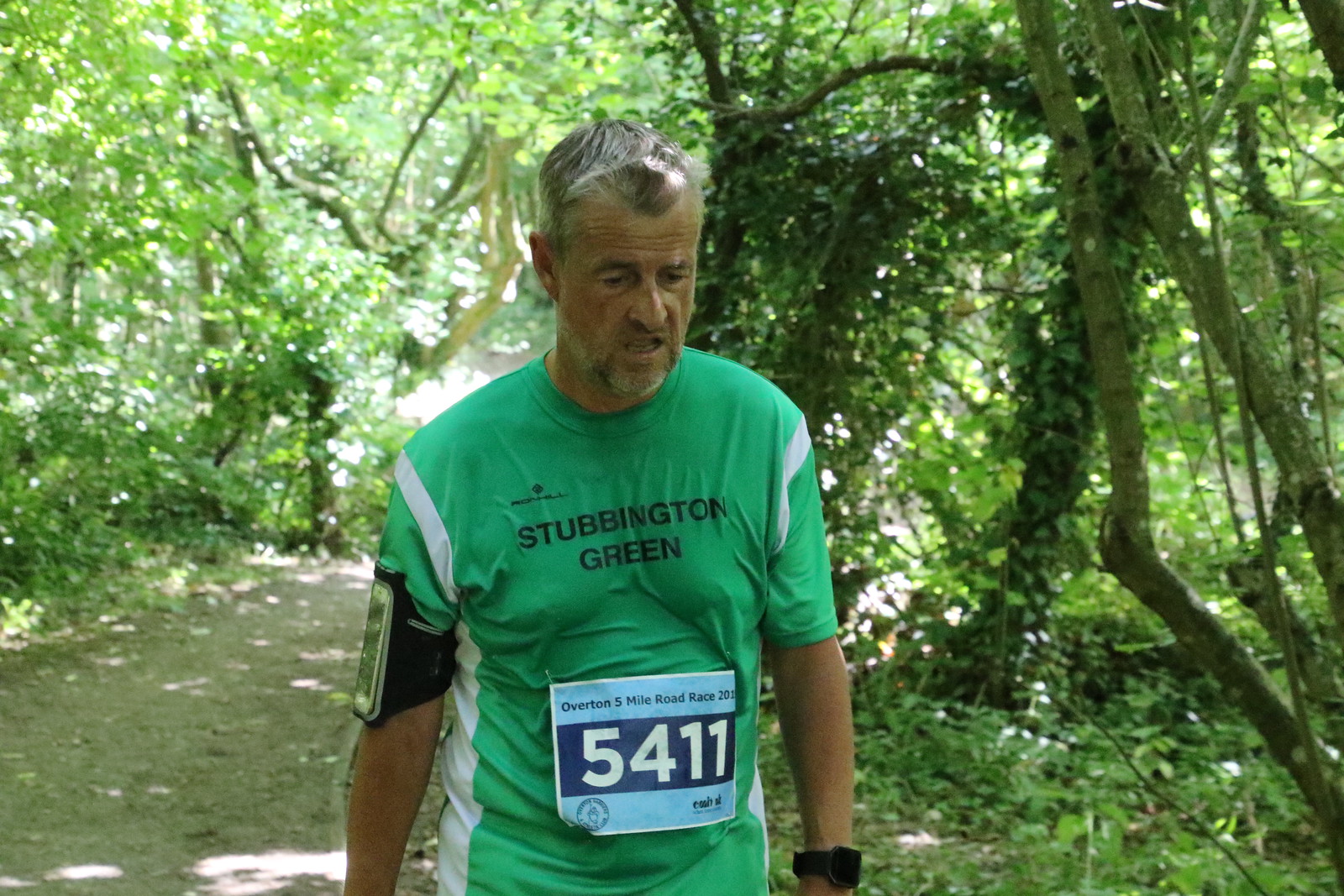In this daylight photo, a weary-looking older Caucasian man, likely in his 50s or late 40s, is participating in a race through a wooded area filled with lush green trees and bushes. The setting is brightened by sunlight streaming through the foliage, creating a serene natural backdrop. Prominently positioned in the center of the image, the man is seen walking slowly along a dirt trail, his tired demeanor evident from his body language and downward gaze. He has short, grey hair, a noticeable goatee, and is dressed in a green jersey adorned with white stripes. His shirt reads "Stubbington Green" and features a logo whose details are unclear. Appended to his shirt at the abdomen is a race bib labeled "Overton 5 Mile Road Race 2001," displaying the number "5411" in white against a blue background, framed by additional logos that are hard to identify. The man's jersey appears drenched in sweat, highlighting his exertion. Additionally, he is equipped with a smartwatch on his left wrist and a mobile phone secured in a holder on his right forearm, underscoring his preparedness for the race.